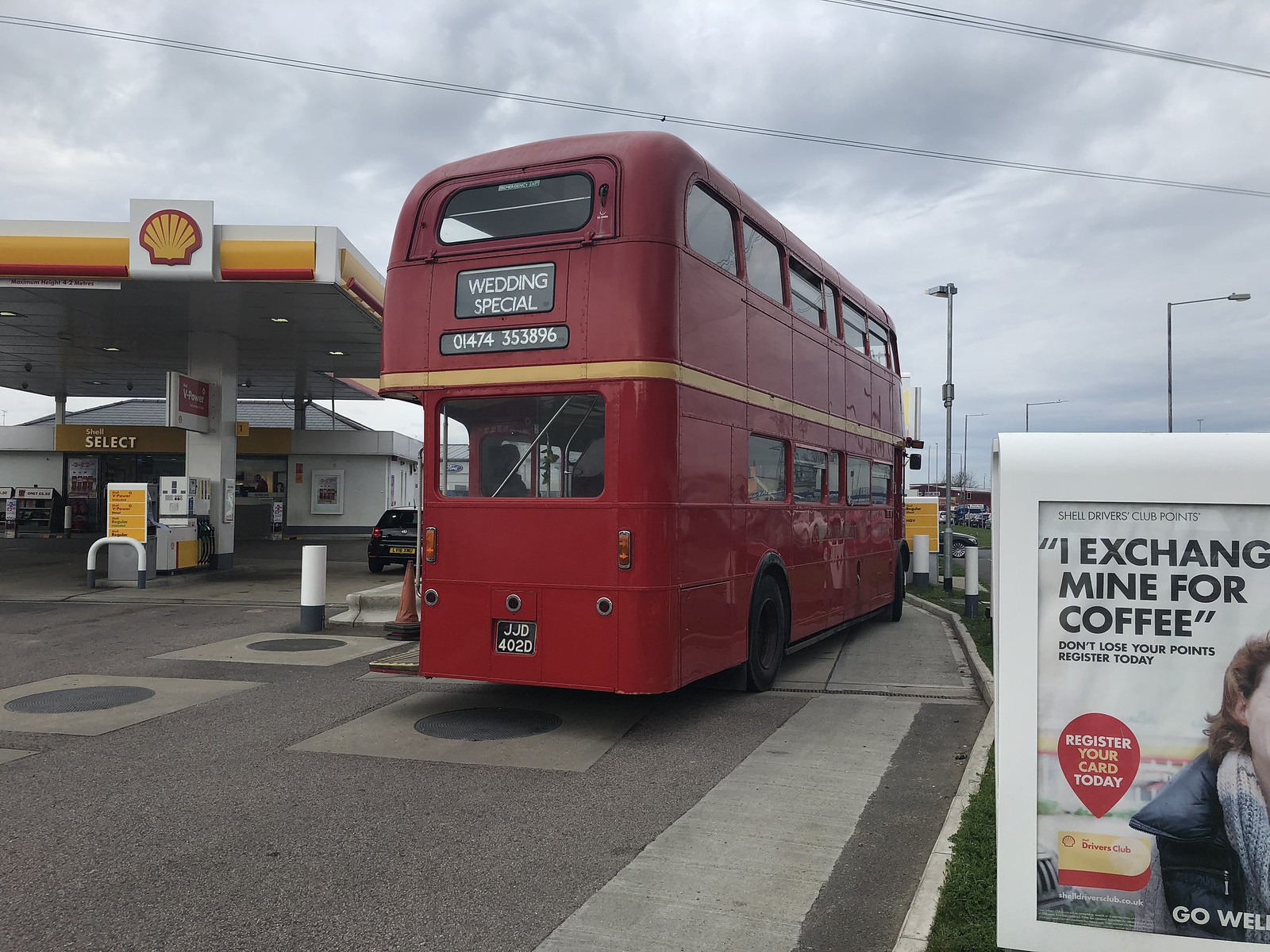The image depicts a classic British red double-decker bus adorned with a "Wedding Special" sign at the back, alongside a contact number, 01474-353-896, and a license plate reading JJ04020. The bus, highlighted by a gold trim separating its two levels, is parked within the vicinity of a Shell gas station, with the station's pumps and yellow Shell emblem visible on the left. The bus rests closely to the curb, making it appear as though maneuvering in this space might be challenging. Another vehicle is seen fueling up nearby. A prominently placed sign in the bottom right corner reads, "Shell Drivers Club Points: I exchange mine for coffee. Don't lose your points. Register today." The sky above is overcast, contributing to the overall cloudy ambiance of the scene. No people are visible in the photograph.